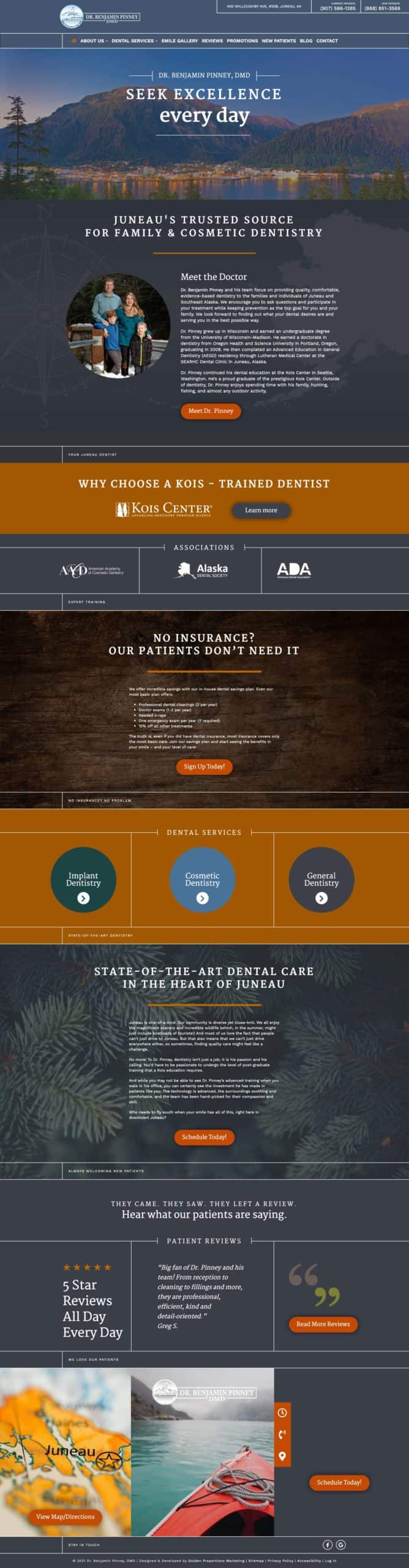This is a detailed caption for the provided image:

The screenshot depicts a webpage that appears quite small and elongated, making the majority of the text difficult to read due to its size. At the top of the page, there is a gray bar featuring a white icon. Directly below this gray bar, large, readable text is present, stating some introductory content. Beneath this text, there is a photograph showing a Caucasian dentist and his family standing outside in a snowy setting.

Following the family photograph, there's a paragraph of text, although it's unreadable in the screenshot due to the tiny font. Below this paragraph, a bold red bar spans the width of the screen. 

Continuing further, there are sequential text sections, each beginning with “it says,” but the specific content remains unclear due to the font size.

At the bottom of the webpage, two small photos are visible: one depicts a map of Juneau, while the other captures a boat peacefully floating in a bay on a misty day. In the lower corner of the screenshot, there is a prominent red oval, possibly highlighting an important feature or button on the webpage.